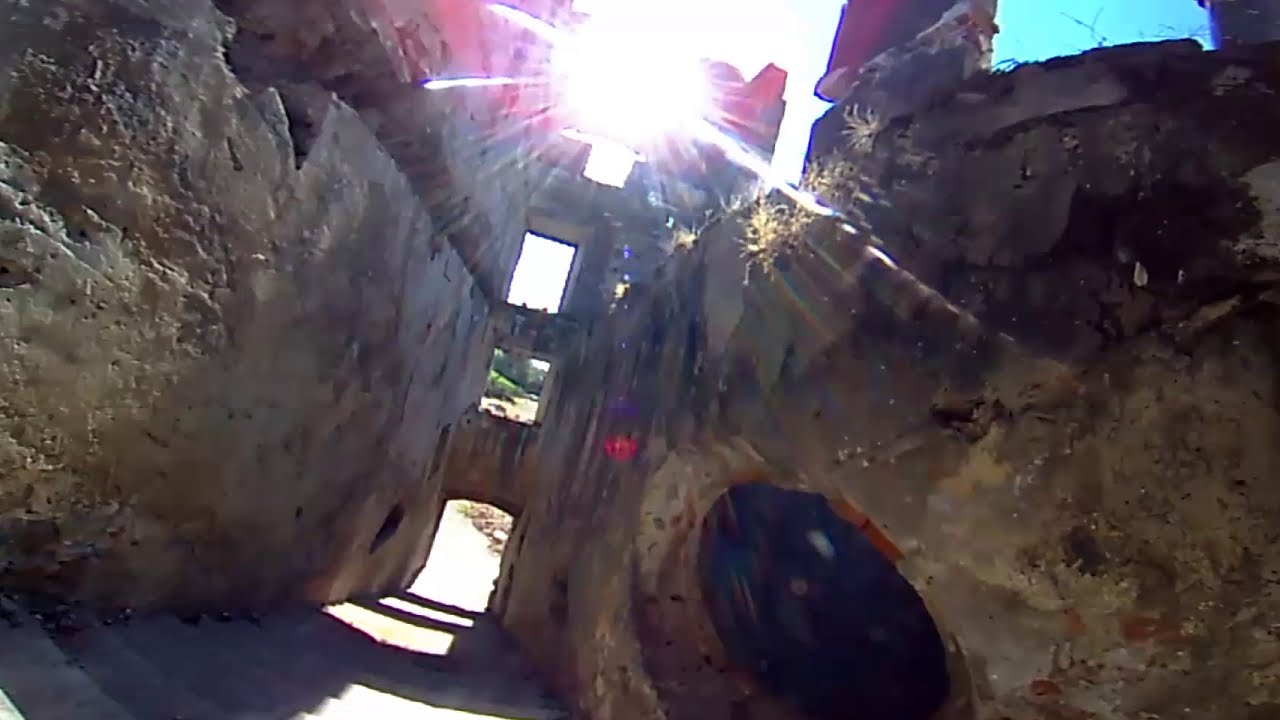This image captures the view from the top of an old, stone stairwell that descends into an entrance of a structure resembling a cave or ancient building. The staircase, made of worn, gray cement, leads down towards an open doorway, framed by tan, chipped stone walls that have aged significantly. To the sides of this passage, built into the structure, are three square openings that let light pour through from outside, highlighting the rocky, handmade nature of the environment. The exterior landscape shows bright sunlight against what appears to be rocks or columns, an indication of the outside world semi-visible through these openings. Above this scene, a clear blue sky stretches across the right part of the image. The photograph, devoid of any text or people, was taken from a perspective that suggests it is mid-day, capturing brilliant sunlight on the old walls and the historical, rustic ambiance of the site. The colors present in the photo include shades of gray, brown, and tan from the stone material, contrasted by the bright blue sky visible through the openings.